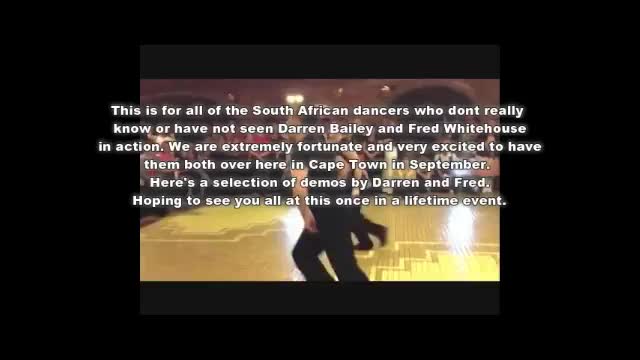The image, framed by a thick black border, showcases a dynamic scene in the middle of a dark background. At the center, several dancers in black short-sleeved shirts and pants are performing on a stage with a gold-toned floor. The floor features a gradient with lighter gold in the upper and back corners. The location appears to be indoors, with a brown building and archways in the background, where an audience is blurrily visible, watching the performance. White text overlays the top half of the image, reading: "This is for all the South African dancers who don't really know or have not seen Darren Bailey and Fred Whitehouse in action. We are extremely fortunate and very excited to have them both over here in Cape Town in September. Here's a selection of demos by Darren and Fred, hoping to see you all at this once-in-a-lifetime event."